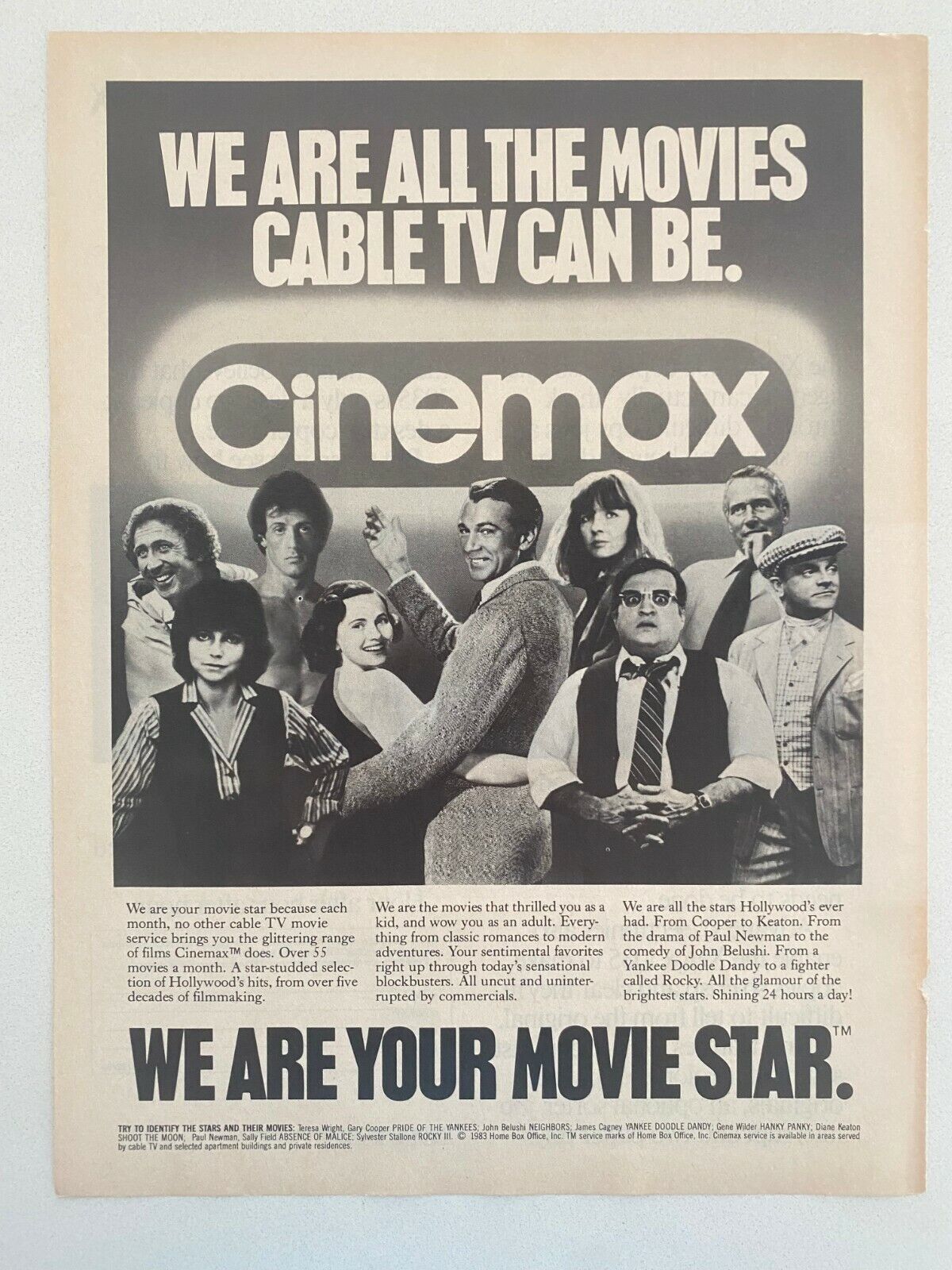The image features a slightly off-white or beige paper from an old newspaper or magazine, pinned against a white wall. Dominating the page is a black and white advertisement with the Cinemax logo. The ad prominently displays the text, "We are all the movies cable TV can be," at the top. Beneath this slogan, there is a collage of nine different people, likely famous movie stars, dressed in vintage outfits from various films. Below the collage, more text appears in a large, bold font that reads, "We are your movie star™," with a trademark symbol over the top right side of the "R."